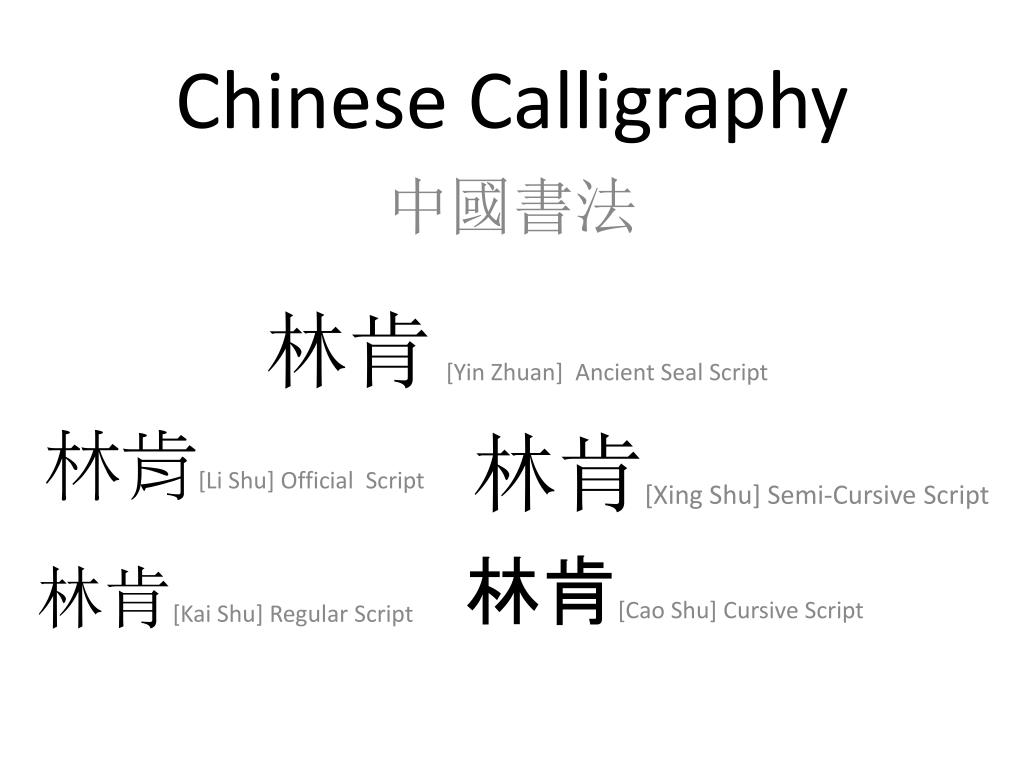The image presents a white background with text prominently featuring "Chinese Calligraphy" in bold black at the top, with the initial letter 'C' capitalized in each word. Directly beneath, there is a row of four gray Chinese calligraphy symbols. Subsequent rows each contain two symbols in black Chinese calligraphy of various styles. The first of these rows is labeled "Yin Zuan Ancient Seal Script" in gray parentheses, the second "Li Shu Official Script," followed by "Xing Shu Semi-Cursive Script," "Kai Shu Regular Script," and finally "Kao Shu Cursive Script." All the Chinese symbols are rendered in dark black ink, while the descriptors are in lighter gray ink, and each descriptive label identifies the script style corresponding to the symbols in that row.